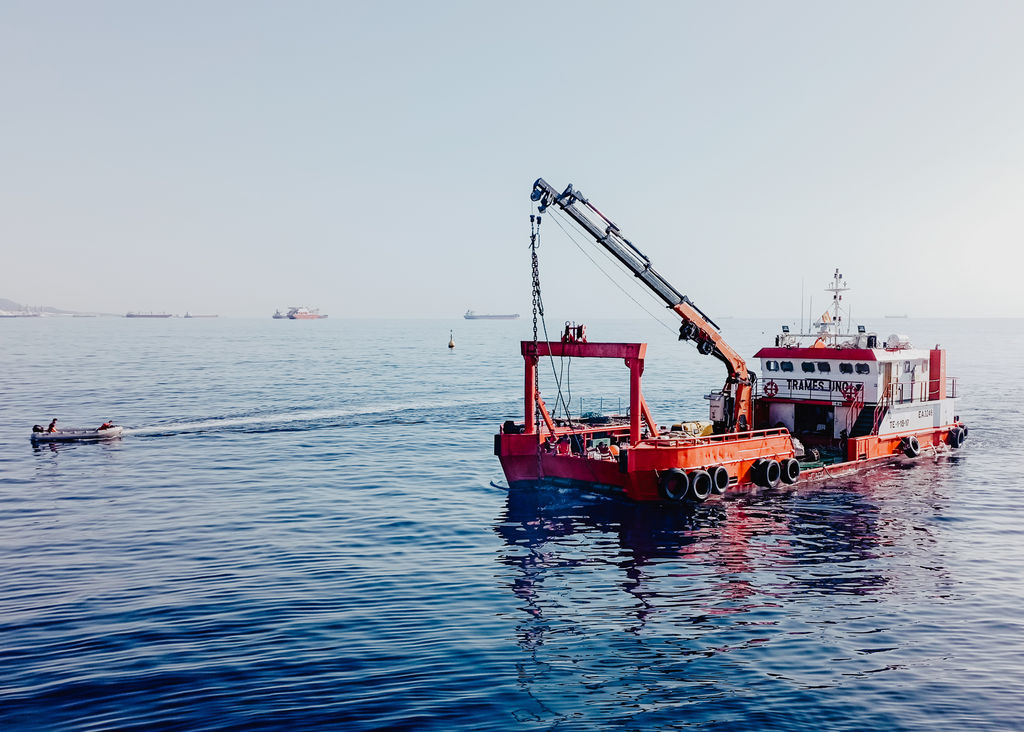This color photograph, taken during the day, showcases a red barge with a white cabin, floating on a vast blue sea. The barge, prominently featuring a large crane with thick chains attached at the back, is equipped with numerous black tires hanging off its sides. The crane, situated toward the rear of the barge, is outstretched with cables hanging down. On the back of the barge, part of the name "T-R-A-M-E-S" can be read, though the rest of the name is obscured by the railing which also holds a life preserver. The barge is absent of visible crew members and is topped with several radio antennas. In the foreground, to the left of the barge, a small motorized boat, which looks like it could accommodate one or two people, is seen moving towards the left. The horizon is dotted with several other ships and boats, implying a bustling maritime scene. The water appears slightly rippled from the movement of the vessels, adding a sense of dynamism to the serene setting.